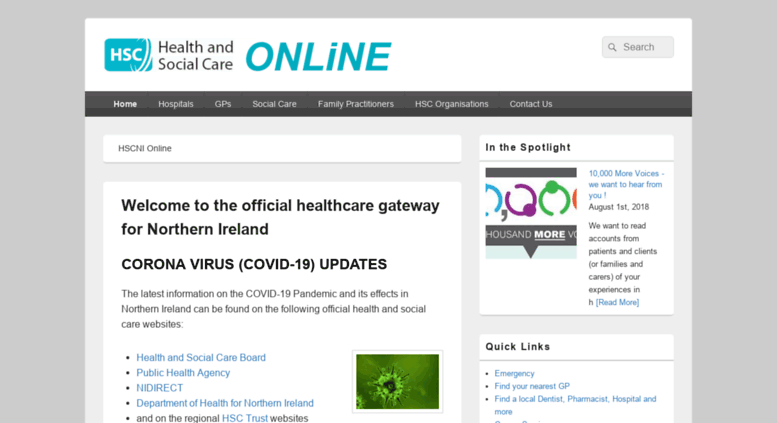This image portrays a clean and structured website interface with a predominantly white background. The theme features a distinct contrast with black text elements. At the top left of the screen, there is a prominent HSC (Health and Social Care) logo set against a blue background with white text. Directly below the logo, the words "Health and Social Care" are displayed in black text, followed by "Online" emphasized in blue text. Positioned on the far right is a search button.

Beneath this top section is a horizontal black navigation bar that spans the width of the screen, containing several white-labeled buttons: Home, Hospitals, GPs, Social Care, Family Practitioners, HSC Organizations, and Contact Us. This bar allows users to access various sections of the site seamlessly.

Directly under this navigation bar is a focused search button, labeled "HSCNI Online." To the left below this button, there's an introductory article titled, "Welcome to the Official Healthcare Gateway for Northern Ireland: Coronavirus (COVID-19) Updates," in bold black text. Beneath the welcome text are various sections about COVID-19, some of which are interactive links indicated by blue-colored text. Adjacent to this text is a green thumbnail image related to COVID-19.

On the right-hand side, there's a "In the Spotlight" section, followed by the headline "Thousands More" and accompanied by small symbols in blue, purple, and green. These symbols have text next to them, the details of which are unclear in the given description. 

Finally, at the bottom of the page, there’s a “Quick Links” section with around five succinct sentence-long links designed for quick navigation to important areas of the site.